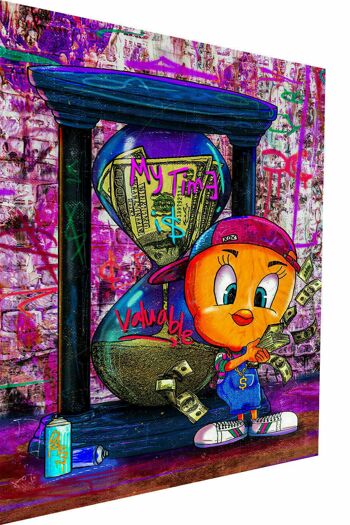The image is a detailed, colorful graffiti artwork featuring Tweety Bird depicted as a gangster. Tweety, with his characteristic yellow feathered face, wears an oversized pair of blue overalls over a green, red, and white striped shirt. He sports a purple and blue backwards cap, white sneakers with green and red stripes, and a conspicuous golden chain with a dollar sign pendant. Tweety is holding a large amount of cash with some bills seemingly flying around him. Behind Tweety, there's a large hourglass with dollar bills at the top gradually trickling down like sand, signifying the message "My time is valuable" with the 'E' in 'time' being backwards and the 'S' in 'is' depicted as a dollar sign. The background features a brick wall covered in various graffiti lines and abstract patterns in pink, white, and brown hues. Additionally, at the bottom left corner, there's a spray can lying on its side, next to another upright can of lighter teal color. This vibrant scene is portrayed as either a framed painting on canvas or wood.